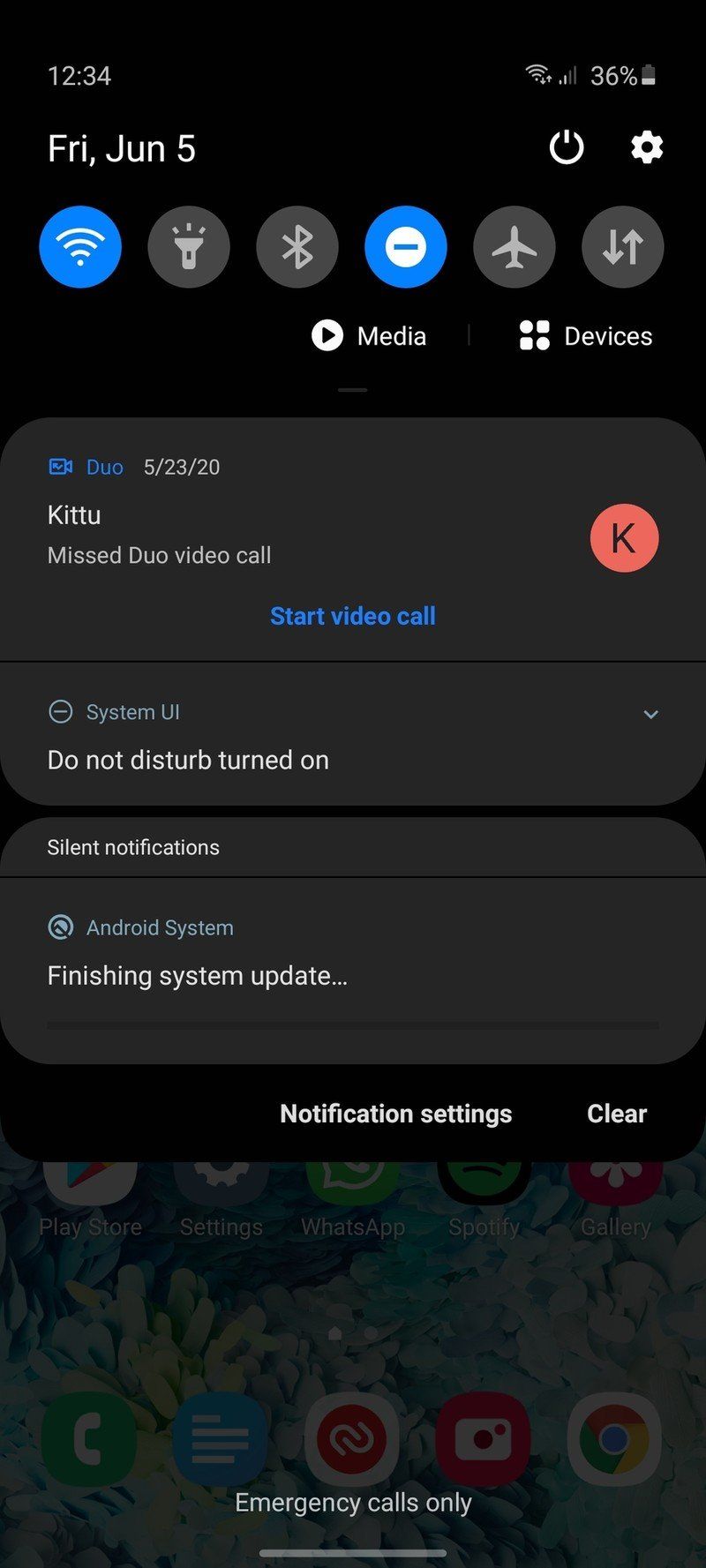This screenshot, likely from a tablet or smartphone, features a predominantly black background. On the top left, a gray text displays "12:34," indicating military time, with "PM" subtly noted. On the top right, there is a Wi-Fi symbol, a cell phone service icon showing 2 out of 4 bars, and a battery icon marked "36%" indicating the battery is a little over a third full. 

Below on the left, bold white text reads "FRI, JUN 5" for Friday, June 5th. At the top, a circle with a line through it signifies power, accompanied by a gear icon for settings. 

Several setting buttons are underneath this: a blue-highlighted Wi-Fi symbol, a gray flashlight symbol, a gray Bluetooth symbol, a dark blue circle with a white center and a blue line, a dark gray circle with a silhouette of a medium gray airplane, and another dark gray circle with gray up and down arrows.

Further down are clickable buttons, including a medium white circle with an overturned black triangle. To the right, there are two circles and two squares, followed by white text that says "devices." A dark gray rectangle features a blue portion resembling a movie camera icon next to the capitalized word "Duo." Below "Duo," in dark gray, the date "5/23/20" is written. In bold gray text, "KTTU" is displayed, followed by "Miss Duo Video Call." A red circle with a black "K" in it is on the right. Below this, a blue text prompts "Start Video Call."

Another dark gray rectangle contains an off-white circle with a line through it, labeled in gray text as "System UI." Bold white text reads "Do Not Disturb turned on," and a larger section beneath indicates "Silent notifications" in white. A gray circle-within-a-circle shows "Android System" next to it, and white text states "Finishing System Update...". 

At the very bottom, in the black bezel, there are options for notification settings and a "clear" option on the right. The center bottom of the screen indicates "Emergency Calls Only."